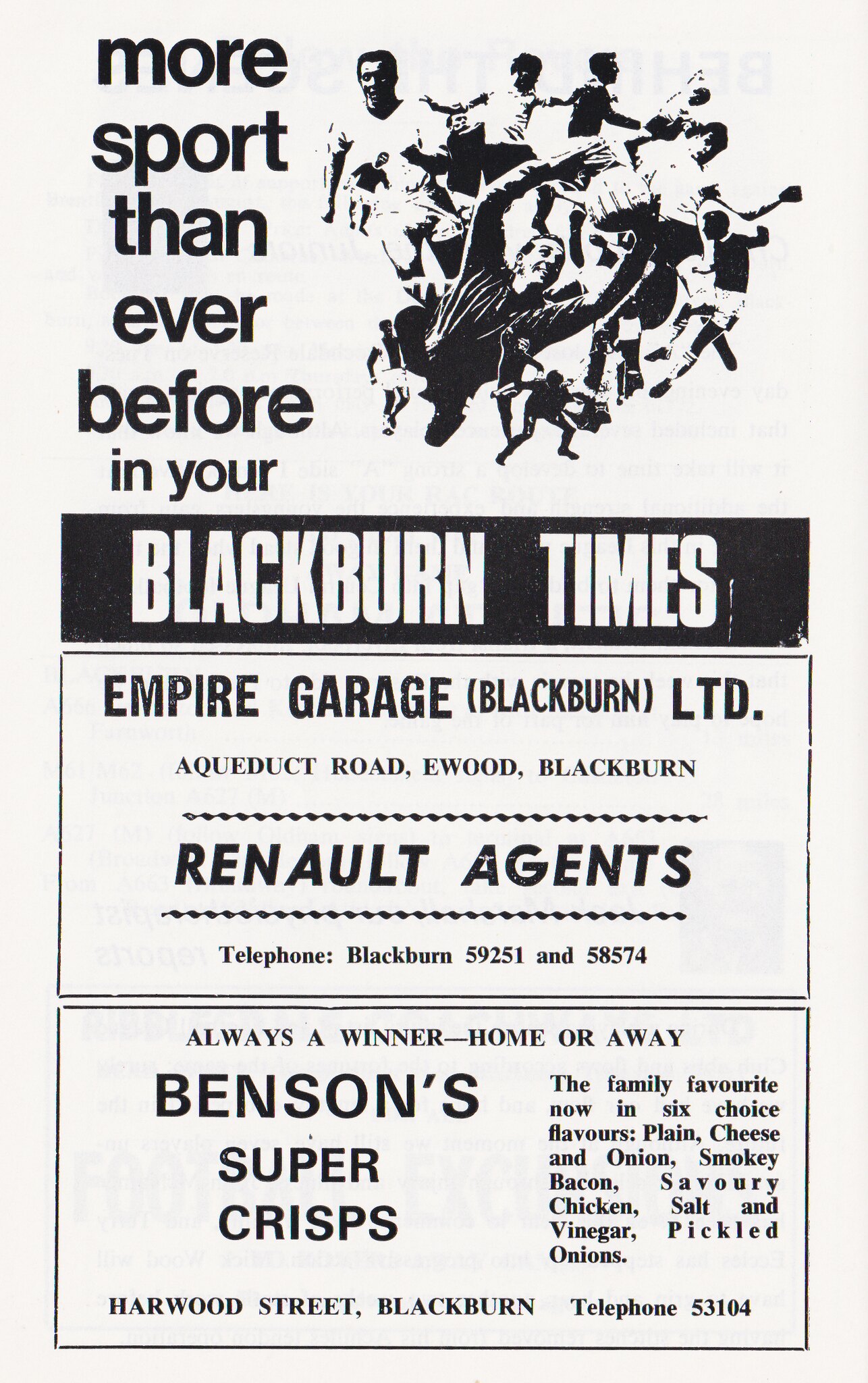This is a detailed description of a poster prominently featuring a local soccer team, presented by the Blackburn Times. The poster, primarily in black and white, showcases an image of the team, illustrated in a caricature style. The headline at the top boldly states, "More Sport Than Ever Before," emphasizing the local sports culture. The publication's logo, "Blackburn Times," is prominently displayed, underscoring its authorship. Additionally, the poster includes information about two key sponsors: Empire Garage, located on Aqueduct Road with contact numbers Blackburn 59251 and 58574, and Benton Super Crisp, situated on Hartwood Street, with the telephone number Blackburn 53104. The imagery and text, albeit simple, convey a strong sense of community support and sports enthusiasm, capturing the local spirit and competitive passion in a nostalgic, almost vintage advertisement ambiance.